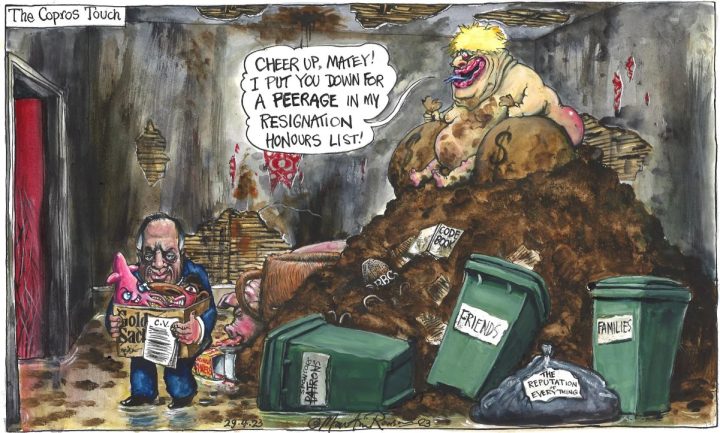This colored political cartoon, formatted as a horizontal rectangle approximately five inches wide by three inches high, showcases a grim, dilapidated room with gray, plaster-stripped walls revealing wooden frames and covered in red marks and brown stains. In the upper left corner on a white background, black text reads "The Kopros Touch." The focal point of the image is a grotesque, naked, obese man with yellow hair and exaggerated facial features, sitting atop a large pile of brown trash. He clutches dirty, brown money bags in each hand. A speech bubble emanates from his mouth saying, "Cheer up, matey, I put you down for a peerage in my resignation honors list." Below the trash mound are three tipped-over green garbage cans labeled "Friends," "Families," and "Patrons," with "Patrons" having been crossed out and replaced with "Sponsors." Additionally, a black trash bag is labeled "The Reputation of Everything." To the lower left, an older balding man dressed in a blue suit carries a box marked "Goldman Sachs," containing pink squids and devilish creatures, as he walks towards a red door, looking back at the viewer. This cartoon is a satirical take on political corruption, embedded within its grimy, visually chaotic setting.